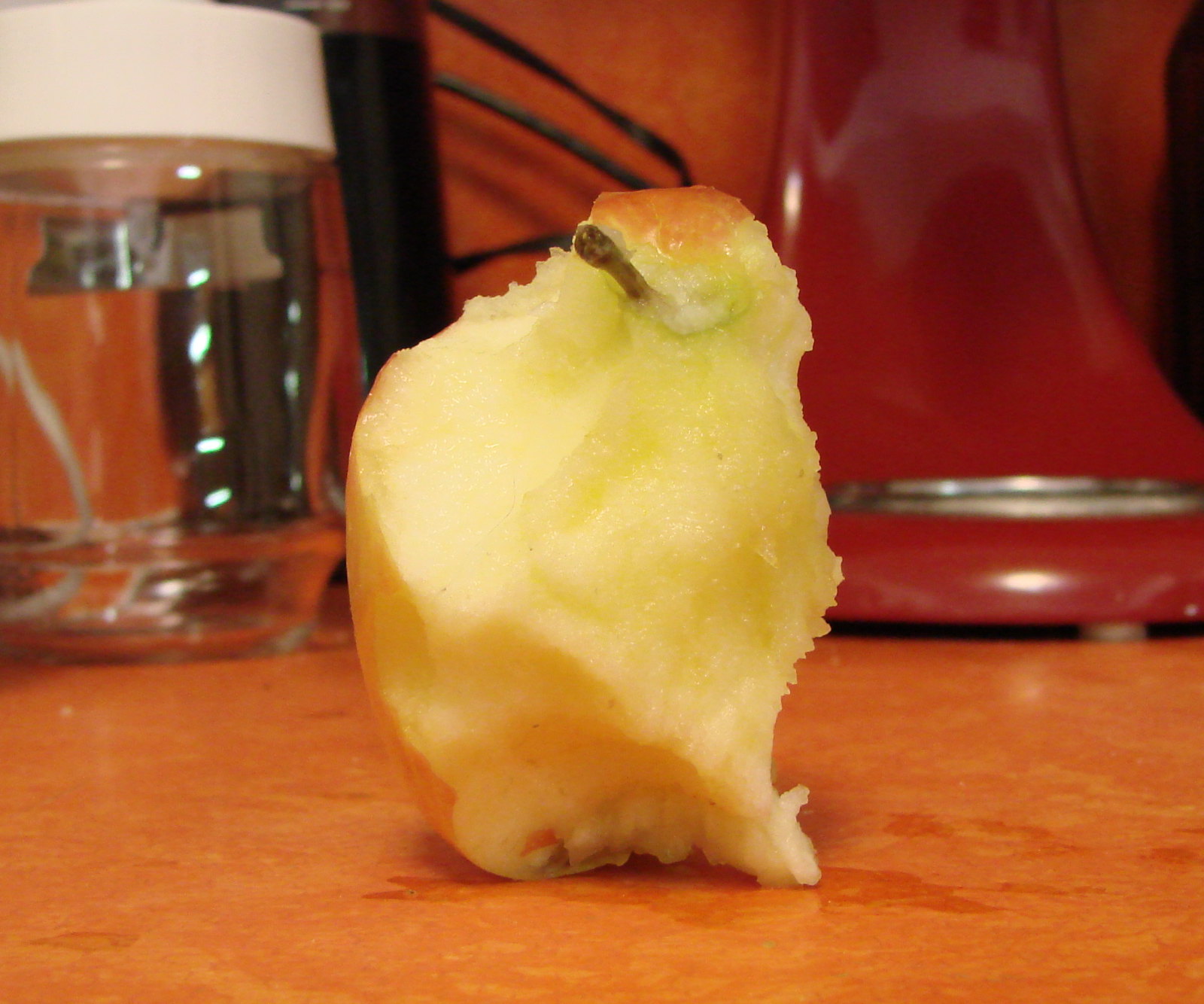A close-up image showcases a partially eaten pear, easily identifiable by its distinct greenish-yellow skin and prominent stem protruding from the top. The fruit's tender, white flesh bears the evident marks of someone's teeth, with irregular angles and indentations where it has been bitten into. A significant portion of the pear remains untouched, indicating it was set down in the midst of consumption.

This pear is resting on a deep amber-colored countertop, whose rich hue contrasts with the fruit's lighter colors. In the background, there is a robust, commercial-quality red base of a blender, equipped with heavy-duty rubber feet for stability. To the left, a clear glass enclosure is visible, which could either belong to this blender or perhaps serve as a coffee maker. The countertop appears slightly soiled, marred by drips and stains likely from the pear itself. Additionally, a tangle of wires and cords runs across the center of the image, adding a touch of everyday kitchen clutter to the scene.